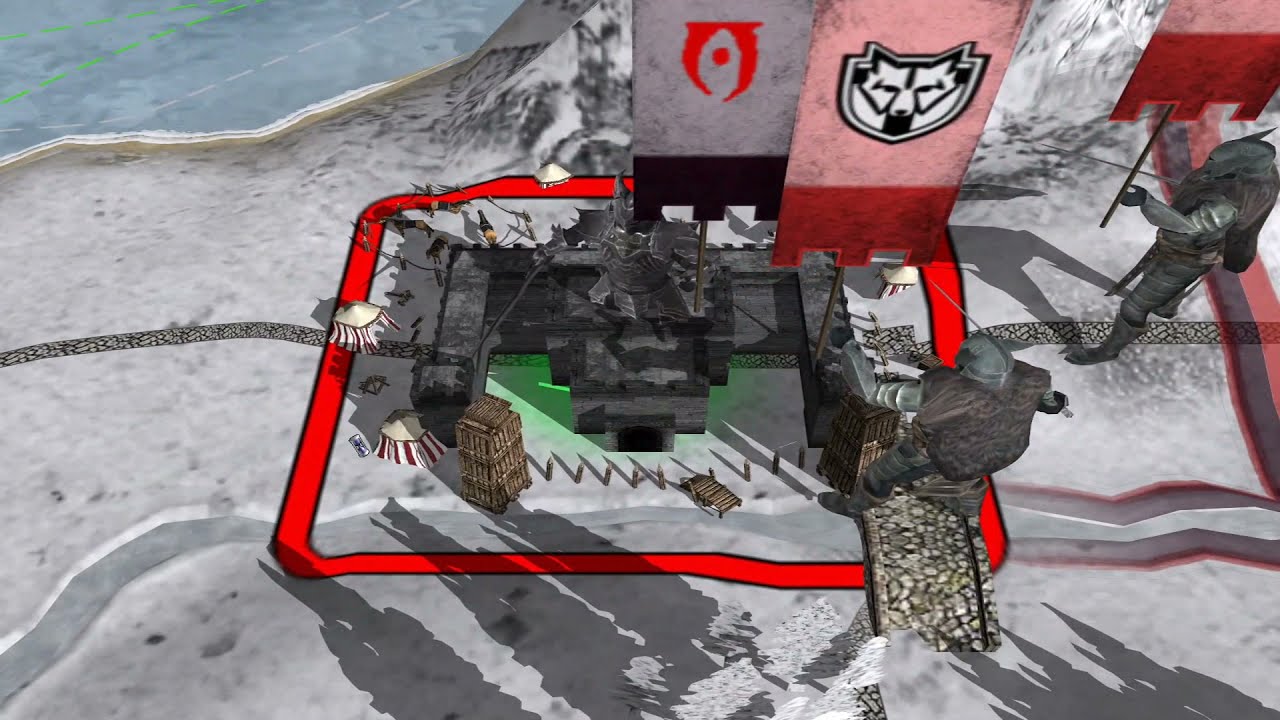In this video game scene, the camera angle, from an elevation of about 15 or 20 feet, captures two humanoid characters clad in full-body armor and helmets that obscure their faces, standing on a grey stone surface. Surrounding them is a scaled-down building resembling a military base with a courtyard. The environment suggests a snowy or wintry setting, with snow-covered ground and a stone mountain towards the upper right. A key detail in the middle of the scene is a red, thick line, possibly indicating a selection or boundary around the base, flanked by two flags. The flag to the right displays a black and white wolf emblem, while the other features a curved symbol with a dot. Nearby, two white and red tents sit outside the base, and a paved road runs through its center. On the far right, a stone walkway bridge extends towards the base, with a character in a grey outfit, appearing to have a wolf's head, walking across it. Additionally, a red banner with a wolf's face and a grey banner with a red symbol add to the militaristic and fantastical atmosphere of this cartoonish, city-building game scene. The oversized armored characters suggest they are giants in relation to the miniature buildings, emphasizing their dominance in the setting.